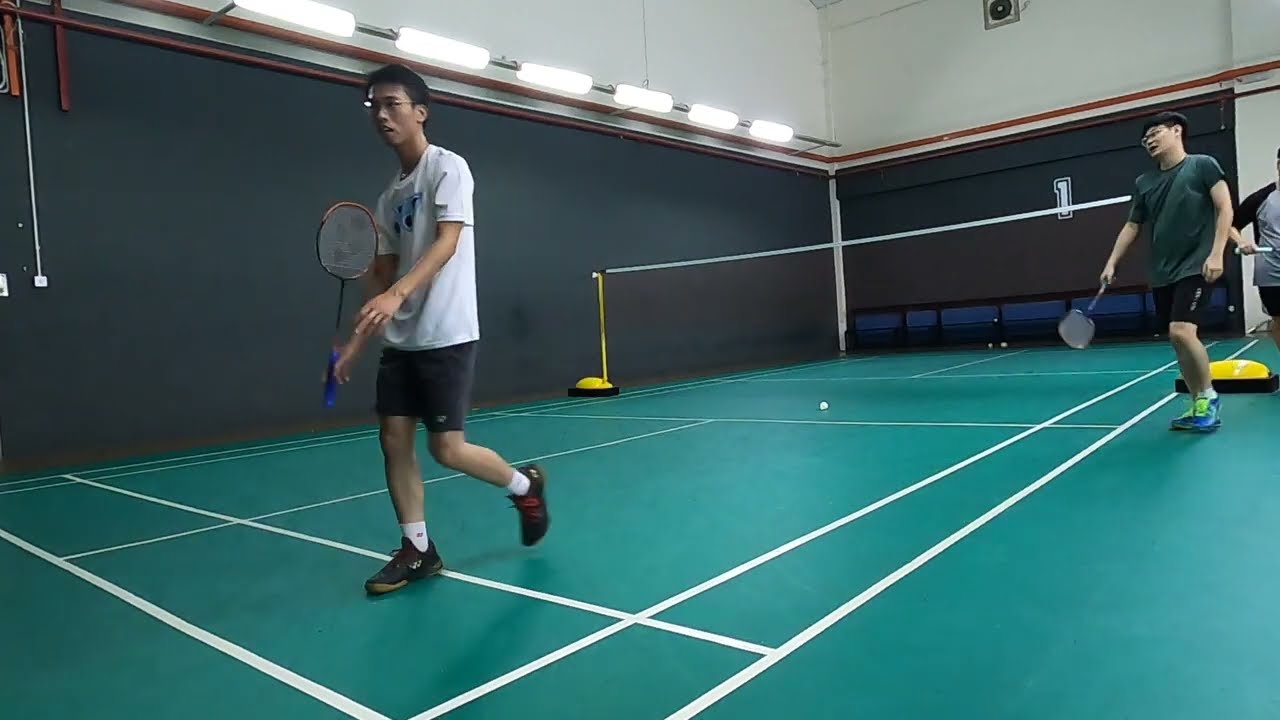The image depicts an indoor pickleball court in a gymnasium or racquet court. The photograph, taken in landscape orientation, captures a bright green court with white striping and a central net anchored by yellow stanchions. The bottom half of the walls are painted dark gray, while the top half is white, with a row of bright lights along the left side.

In the scene, two young men, both appearing to be about 20 years old and of Asian descent, are captured. On the left side of the image, a man wearing a white t-shirt, black shorts, white socks, and black sneakers is walking towards the left, looking at the camera. He holds a pickleball racket in his right hand and sports black eyeglass frames with black hair. To the right, near the midpoint of the court, another young man is visible, wearing a gray shirt, black shorts, and blue and gray sneakers. He also holds a racket in his right hand and is looking towards the left. Part of a third man's torso and arm is visible on the far right, indicating the presence of another player. In the background, the court is marked as number one, and some seats can be seen, suggesting it might have been a doubles game. The image captures a moment of realism and active engagement within the indoor sports facility.